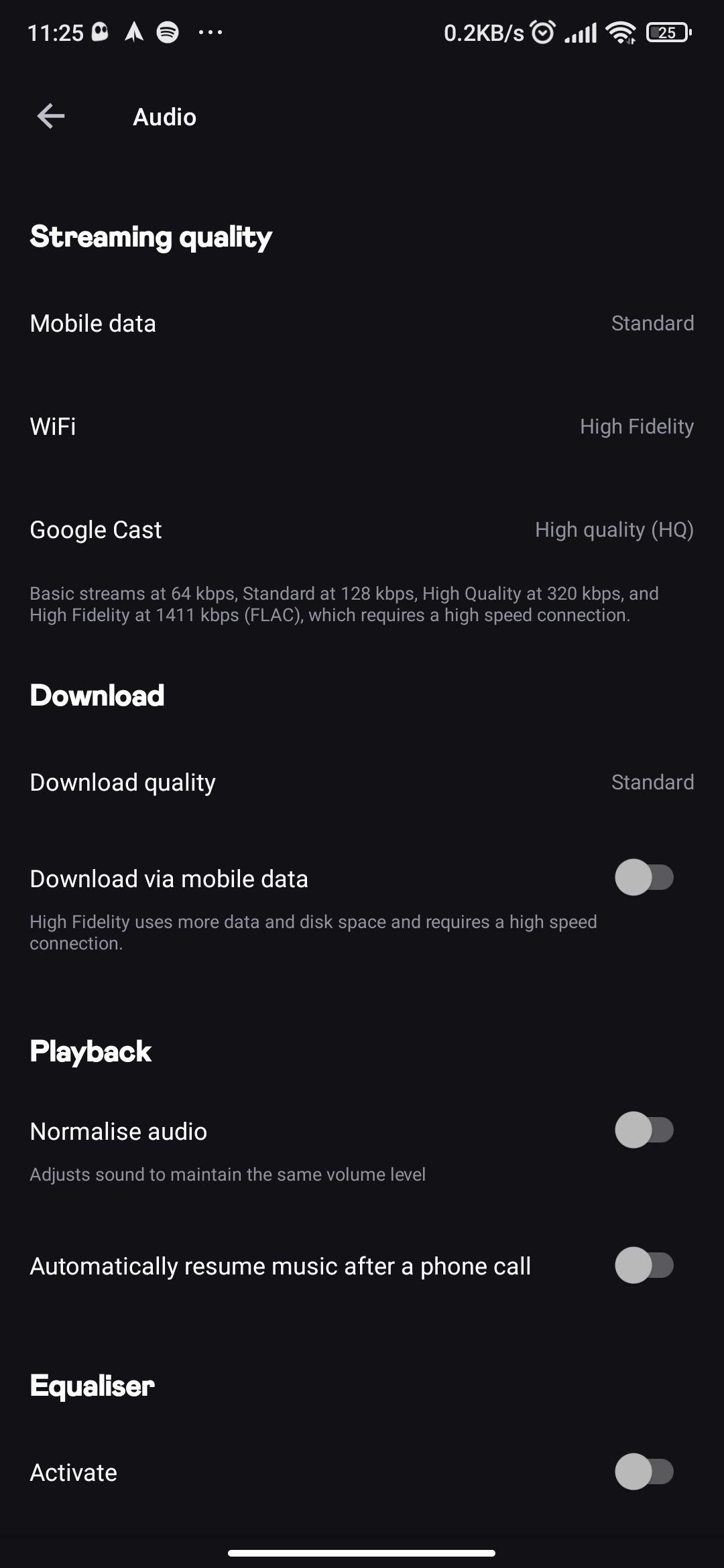The image features a smartphone screenshot captured at 11:25, as indicated by the time display at the top of the screen. The status bar shows several standard icons: a white circle resembling a mail or envelope icon, an active alarm, full carrier signal strength, Wi-Fi enabled, and a battery level at 25%.

The main content of the screenshot is the audio settings menu. At the top-left corner, a white arrow allows navigation to the previous screen. Below that, the audio settings detail various streaming and playback options:

- **Streaming Quality for Mobile Data**: Set to standard.
- **Wi-Fi**: Set to high fidelity.
- **Google Cast**: Set to high quality (HQ).

A detailed breakdown of streaming quality options is provided:
- Basic streams at 64 kbps.
- Standard streams at 128 kbps.
- High quality streams at 320 kbps.
- High fidelity streams at 1411 kbps, which require a high-speed connection.

Two main sections are highlighted:

- **Download**: This section is bolded, indicating it’s currently selected. The download quality is set to standard, and downloading via mobile data is turned off.
- **Playback**: Also bolded, this section highlights that 'Normalize Audio' is turned off and 'Resume Music After a Call' is also off.

Overall, the image provides a comprehensive look at the user's current audio settings on their smartphone.